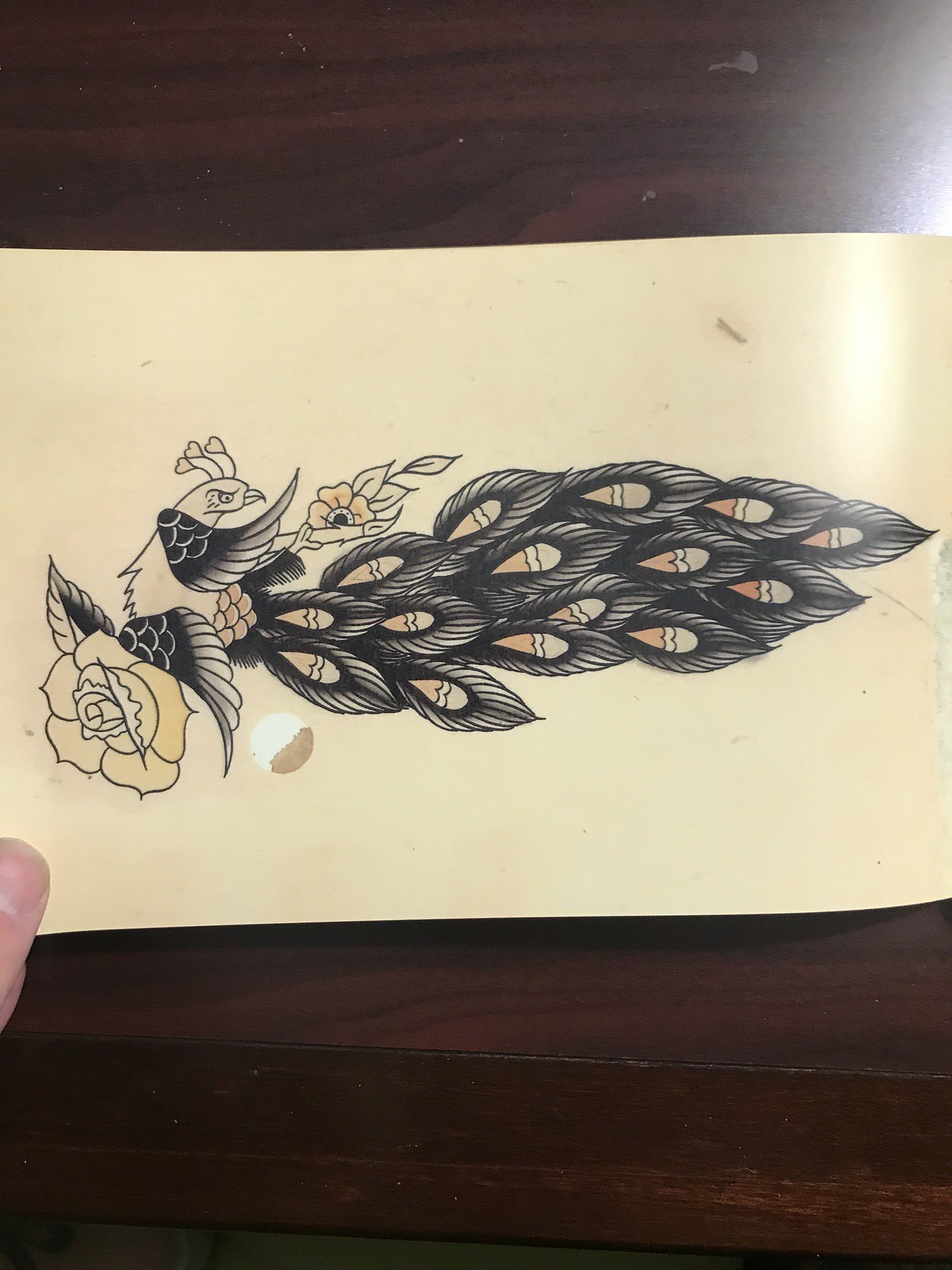A meticulously detailed drawing of a peacock adorns a piece of white, eggshell-colored paper, oriented horizontally. The vibrant artwork captures a peacock perched elegantly on a rose, with its elaborate tail feathers gracefully extending towards the right side of the image. A person's thumb is visible on the left, holding the paper steady. In the background, the texture of a brown table subtly contrasts with the artwork, allowing the peacock's intricate details to take center stage.